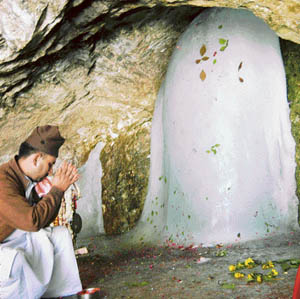In a dimly lit cave with rough, natural light-brown rock walls, a man kneels on the ground, his body turned slightly to the side as he bows in deep prayer. His head is bent low, eyes closed, and hands clasped together just in front of his face. He wears white, baggy trousers and a brown coat, complemented by a brown, floppy knit cap that sits slightly oversized on his head. The platform on which he kneels is obscured, blending into the rocky cave floor. 

In front of him, a ghostly white mound—resembling frozen flow ice—rises from the ground, adorned with scattered leaves and surrounded by a delicate ring of yellow flowers, perhaps an offering. To the right, a small frozen waterfall cascades down, its icy flow decorated with additional flowers and leaves. The cave's entrance bathes the scene in light, contrasting the shadows that mark the upper portions of the cavernous space. Overall, the image is serene yet somber, capturing a solitary moment of reflection and reverence.